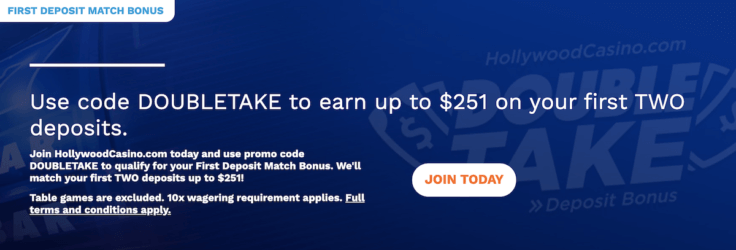This image is a screenshot, presumably taken from a computer, and appears to be from the top advertisement section of a website. The top left corner features a small, white area with rounded corners, containing the text "First Deposit Match Bonus" in light blue. The majority of the background is dark blue with overlaying text.

In the background, the text "hollywoodcasino.com Double Take Deposit Bonus" can be seen. Superimposed on this, in white font, is a promotional message: "Use code DOUBLETAKE to earn up to $251 on your first two deposits. Join hollywoodcasino.com today and use promo code DOUBLETAKE to qualify for your first deposit match bonus. We will match your first two deposits up to $251." Additional details state that table games are excluded, a 10-times wagering requirement applies, and full terms and conditions are available via an underlined hyperlink.

To the right of this text is a white button with rounded corners that says "Join Today" in orange. Above the promotional code mention, a white line about an inch long is visible. The background implies a computer interface, though it’s not distinctly clear.